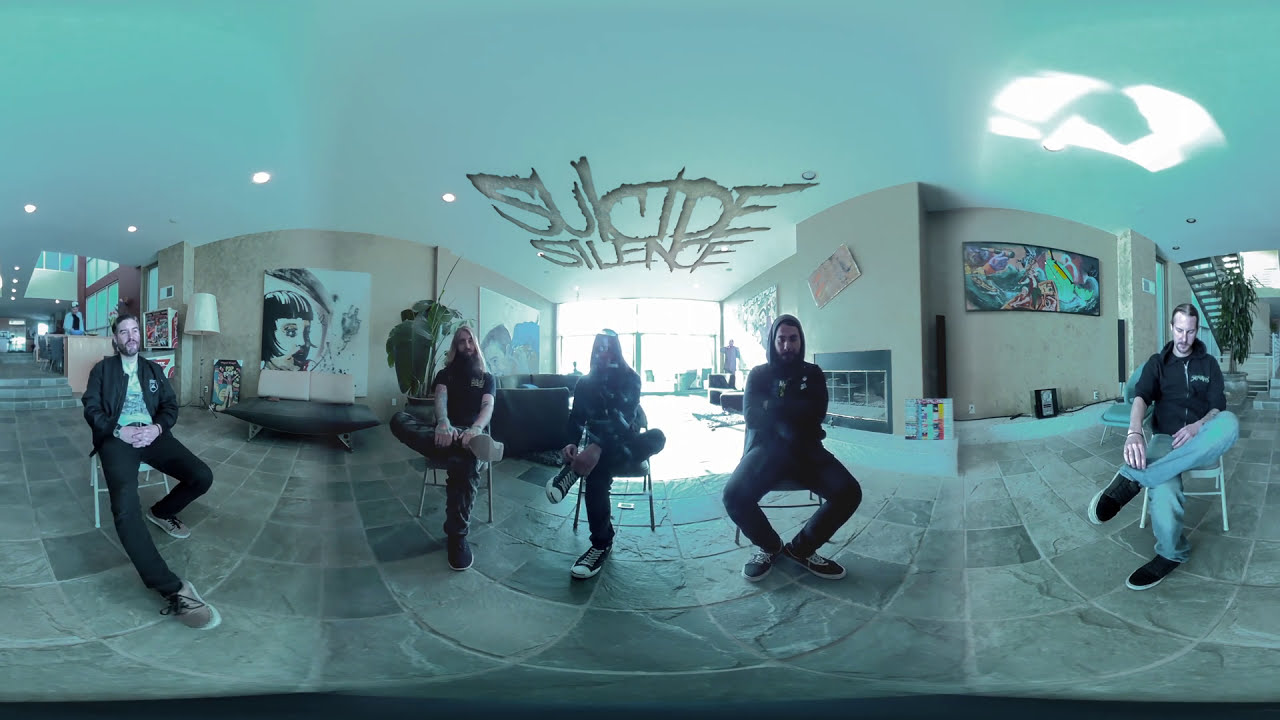The photograph depicts a wide-angle, panoramic view of an upscale indoor setting, possibly an art gallery or living room. Five individuals, who predominantly appear to be men with long hair, casual attire, and facial features suggesting they are musicians, are seated in a linear arrangement on straight-back chairs. Centered above them on the ceiling, in scraggly, knife-like font, the words "Suicide Silence" are prominently displayed, indicating it could be the name of a band.

The room boasts modern art on beige walls, a stone-patterned floor, and numerous plants and lamps dispersed throughout the space. The ceiling is a grayish-blue hue with recessed lighting, enhancing the bright, natural light streaming in from a large window positioned behind the central figures, which causes significant backlighting and partially obscures the middle individual.

To the left and right of the scene, there are staircases leading to a second story. The men are dressed in dark, casual outfits, including jeans, t-shirts, hoodies, and sneakers. They exhibit serious, deadpan expressions, with various poses ranging from crossed legs to arms folded over chests, suggesting a somber or contemplative mood. The overall ambiance is enriched by modern decor and the juxtaposition of contemporary art and natural elements like plants, creating a sophisticated yet relaxed atmosphere.